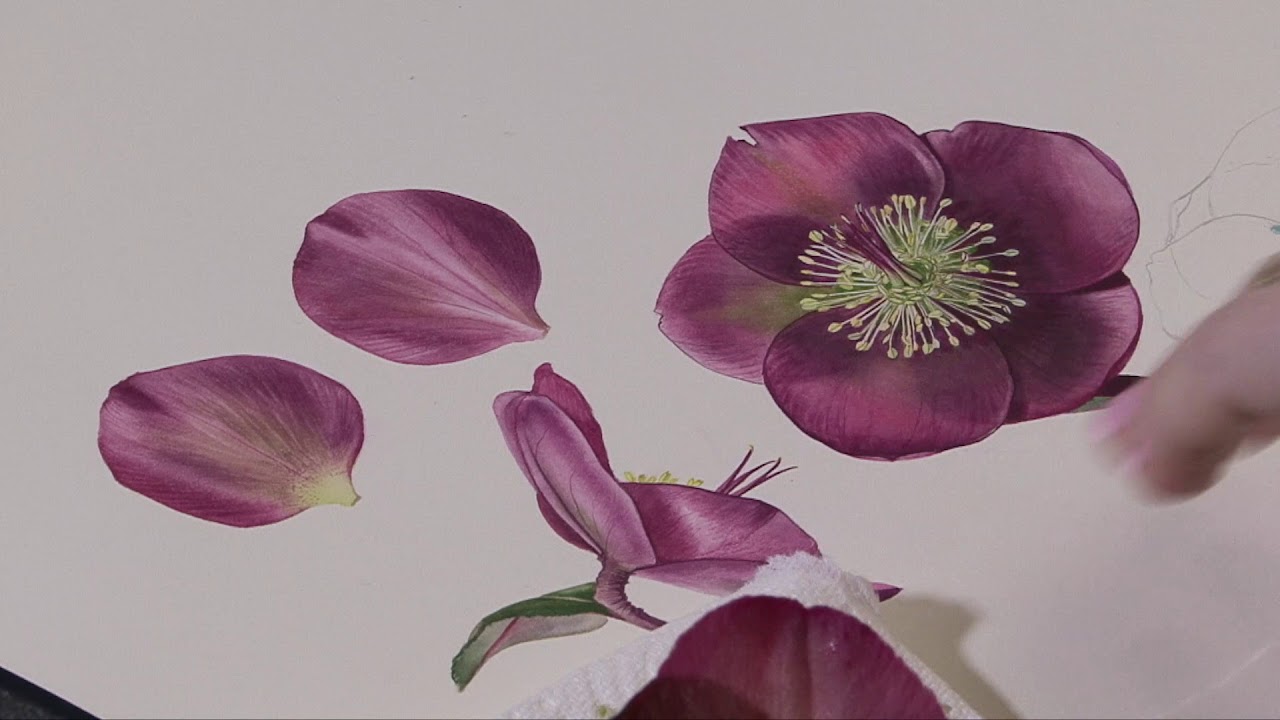The image depicts an intricately detailed illustration or painting of a purple Hellebore flower on white paper. The artwork appears to be in progress, as evidenced by the sketch marks of flower petals visible on the right edge and a blurry fingertip suggesting recent activity. The central focus is a fully painted Hellebore flower with five dark purple petals accented by even darker lines and a vibrant green stamen with yellowish-white pollen strands. To the left, two individual petals are meticulously painted, showcasing their dark purple hue with lighter edges. Below these, a side view of the flower reveals an elegantly curved green leaf beneath it. The Hellebore's petals, both individually and in full bloom, display intricate details with their slight pointy tips and delicate connection to the stem. The composition captures the ephemeral beauty of the flower in both its sketch and painted forms. Just below the flower, an indistinct cloth with floral patterns adds texture to the artistic scene.